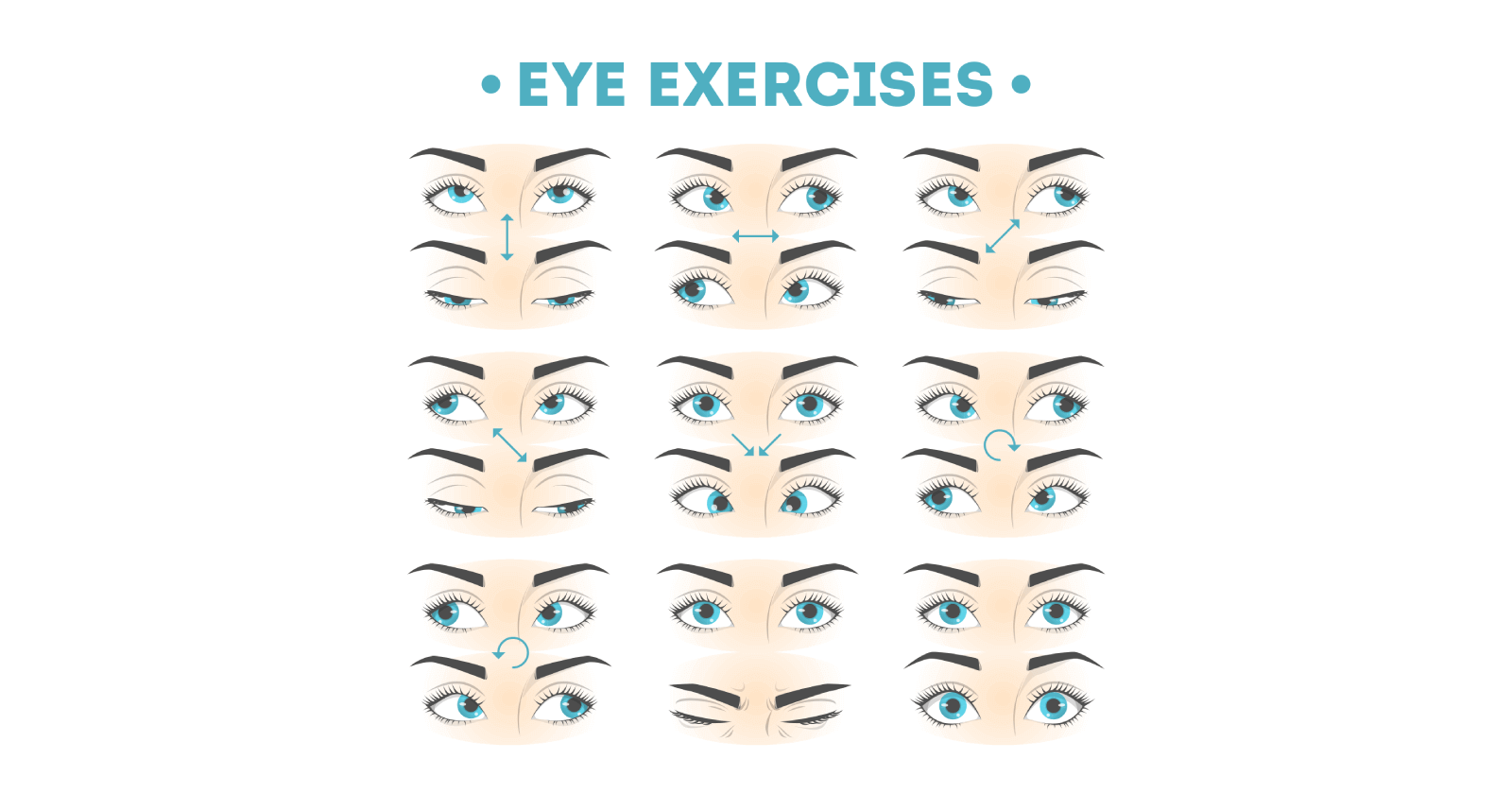This image, designed as a poster, depicts nine distinct eye exercises against a white and blue background. The title "EYE EXERCISES" is prominently displayed at the top in capitalized blue font, flanked by two blue periods. Each exercise features illustrations of eyes with tan skin, black eyebrows, and blue irises. 

Starting from the top left and moving to the bottom right, the exercises are categorized as follows: 

1. **Vertical Eye Movement**: One set of eyes looks upward, and another looks downward, with a vertical arrow showing the movement up and down.
2. **Horizontal Eye Movement**: Eyes are illustrated looking left and right, with a horizontal arrow indicating the side-to-side motion.
3. **Right Diagonal Eye Movement**: Eyes move diagonally from the bottom left to the upper right, as depicted by a diagonal arrow.
4. **Left Diagonal Eye Movement**: Similar to the previous, but in the opposite direction, moving from upper left to bottom right with a diagonal arrow.
5. **Inward Eye Movement**: Eyes are shown looking inward diagonally with arrows pointing from top right to bottom left and top left to bottom right.
6. **Eye Cross**: Eyes start off looking straight ahead and then cross inward, indicative of focusing on a close object.
7. **Circular Eye Movement**: Depicted by a circular arrow, eyes start looking right and then roll around in a circular motion.
8. **Curved Eye Movement**: Eyes move in a curved path from left to right, denoted by a curved arrow.
9. **Eye Open/Close**: Two sets of eyes are shown, one open and the other closed, without any directional arrows, indicating a simple open-close exercise.

Each visual is detailed with black eyebrows and blue irises, serving as a comprehensive guide for performing these eye exercises effectively.